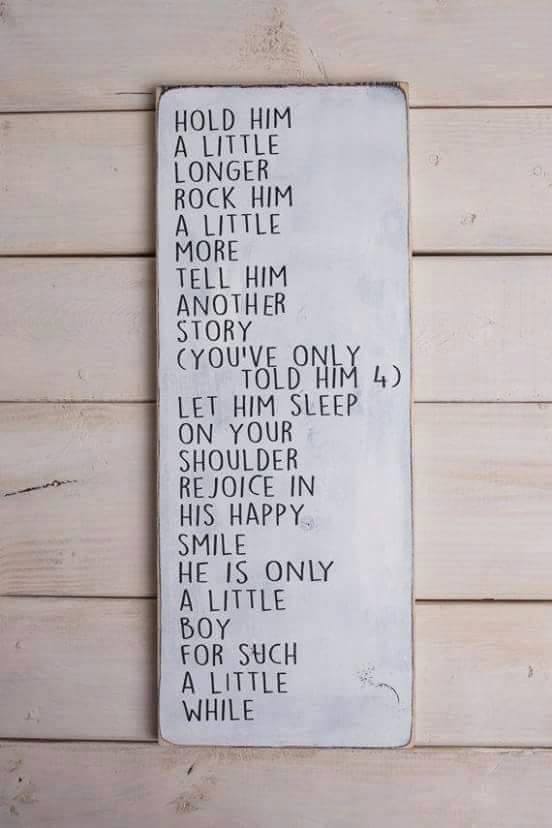The image features a weathered, creamy beige wooden siding, possibly the exterior of a house, with six horizontal planks visible. Centered on this rustic backdrop is a tall, rectangular sign with a whitish-gray background and bold black text in all capital letters. The sign reads: "HOLD HIM A LITTLE LONGER, ROCK HIM A LITTLE MORE, TELL HIM ANOTHER STORY (YOU'VE ONLY TOLD HIM FOUR), LET HIM SLEEP ON YOUR SHOULDER, REJOICE IN HIS HAPPY SMILE, HE IS ONLY A LITTLE BOY FOR SUCH A LITTLE WHILE." The sign is slightly worn and hangs evenly in the middle of the image, adding a touch of sentimental charm to the already quaint setting.